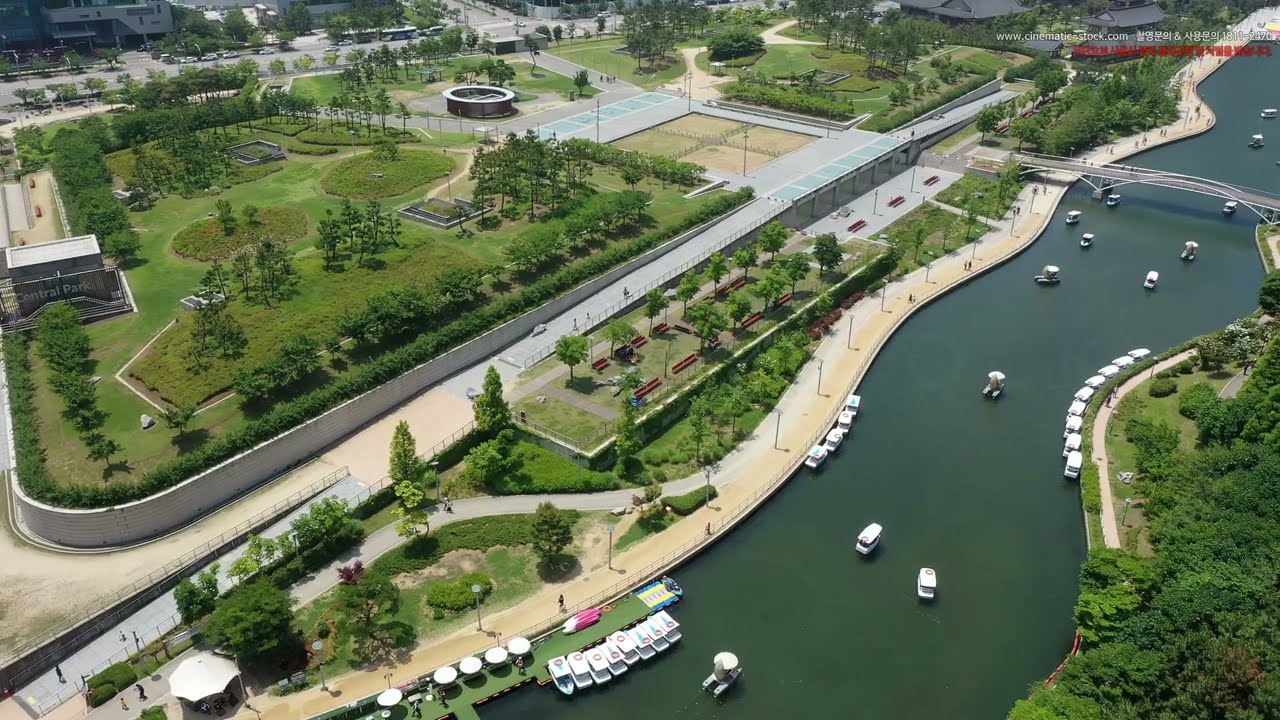The aerial image provides a captivating overhead view of an urban park bisected by a curving river, which flows from the bottom center towards the upper right-hand corner. The river, appearing almost green, is dotted with several fan boats. Adjacent to the water, both sides are lush with green grass, shrubs, and trees. A notable feature is a pier stretching towards the water with light-colored pathways and a few people walking along it. A bridge spans across the river, connecting the areas of greenery and the pier.

To the right of the river, dense green tree clusters intensify the natural scenery. The left side showcases a transition from parkland to urban, starting with green spaces and then incorporating roads and small buildings near the river. Further left, the landscape becomes more urbanized with the presence of a tall building and a large parking lot in the upper left-hand corner.

Additional elements include text in the upper right-hand corner emblazoned with "www.cinematicdeckstock.com" accompanied by Asian characters. Overall, the image expertly captures the harmony of green park areas with their trees and grass, interspersed with urban elements, anchored by the central graceful bend of the river.